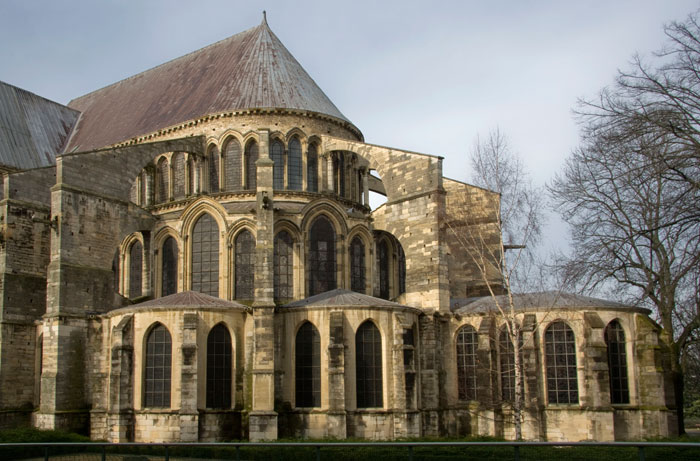This photograph captures an imposing, distressed manor house with a distinct gothic vibe, set against a backdrop of a gray, cloudy sky. This yellowish, golden-tan, and brown-brick building spans three levels, with intricate architectural details that merge elements of a cathedral and a manor house. The ground floor features three circular rooms adorned with stone pillars, while the second floor boasts a large circular room with several tall, arched, cathedral-like windows filled with dark latticework. Another level above mirrors this design, crowned by a brown, rusted metal roof that ascends to a point. The building sits behind a fence bordered by shrubbery, adding to its enigmatic charm. To the right of the structure, bare trees with no leaves enhance the sense of desolation and age. The entire scene is devoid of people, emphasizing the eerie, timeless quality of this grand, weathered edifice.